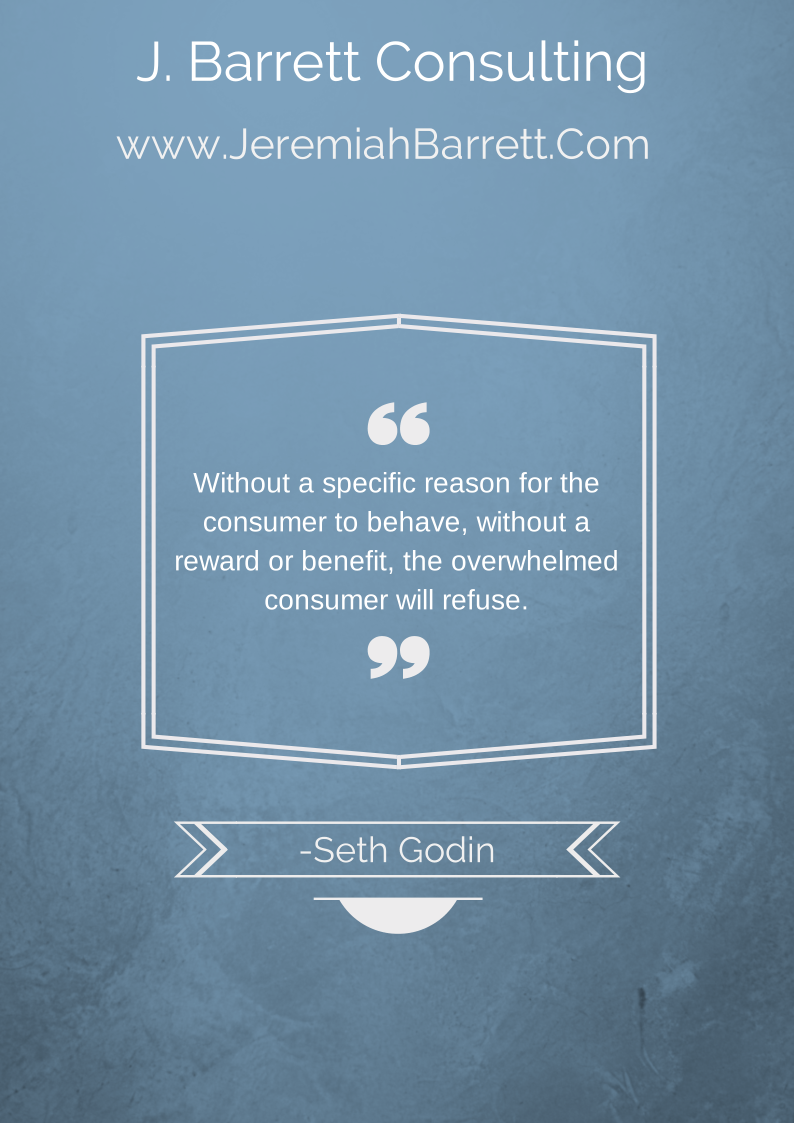The image is a minimalistic poster set against a gradient bluish background that transitions from lighter blue at the top to darker blue at the bottom. At the top of the poster, in white text, it reads "J. Barrett Consulting" with the web address “www.jeremybarrett.com” directly below it. The initials "J," "B," and "C" in "J. Barrett Consulting" are capitalized. In the center of the poster, enclosed within a white bordered square, is a quote also in white text: "Without a specific reason for the consumer to behave, without a reward or benefit, the overwhelmed consumer will refuse." This quote is framed by white quotation marks at both the top and bottom. Below the quote, another white-bordered box contains the name "Seth Godin," with decorative white arrows pointing towards it and a small line featuring a half-circle beneath it. The overall design uses simple, clean lines and focuses on the contrast between the white text and the blue background to deliver a professional and inspirational message.